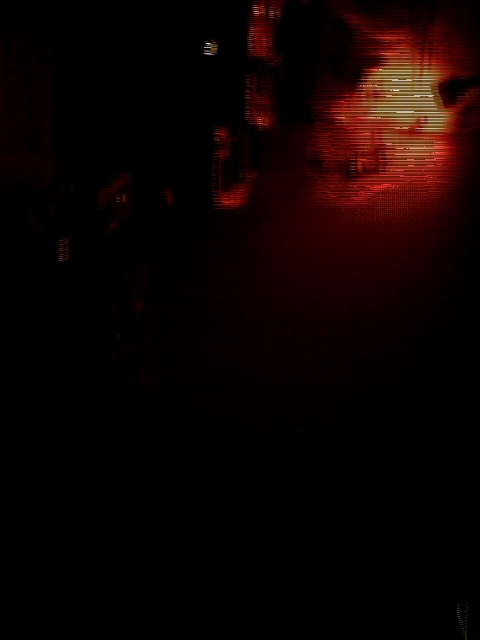The image is extremely blurry, rendering most details indistinguishable. Dominated by deep blacks, the only notable feature is a warm, soft red light in the top right corner. This light could possibly be a lamp, though its exact form is unclear. There are also faint horizontal lines running across the image, but these provide no additional clarity to the overall scene.